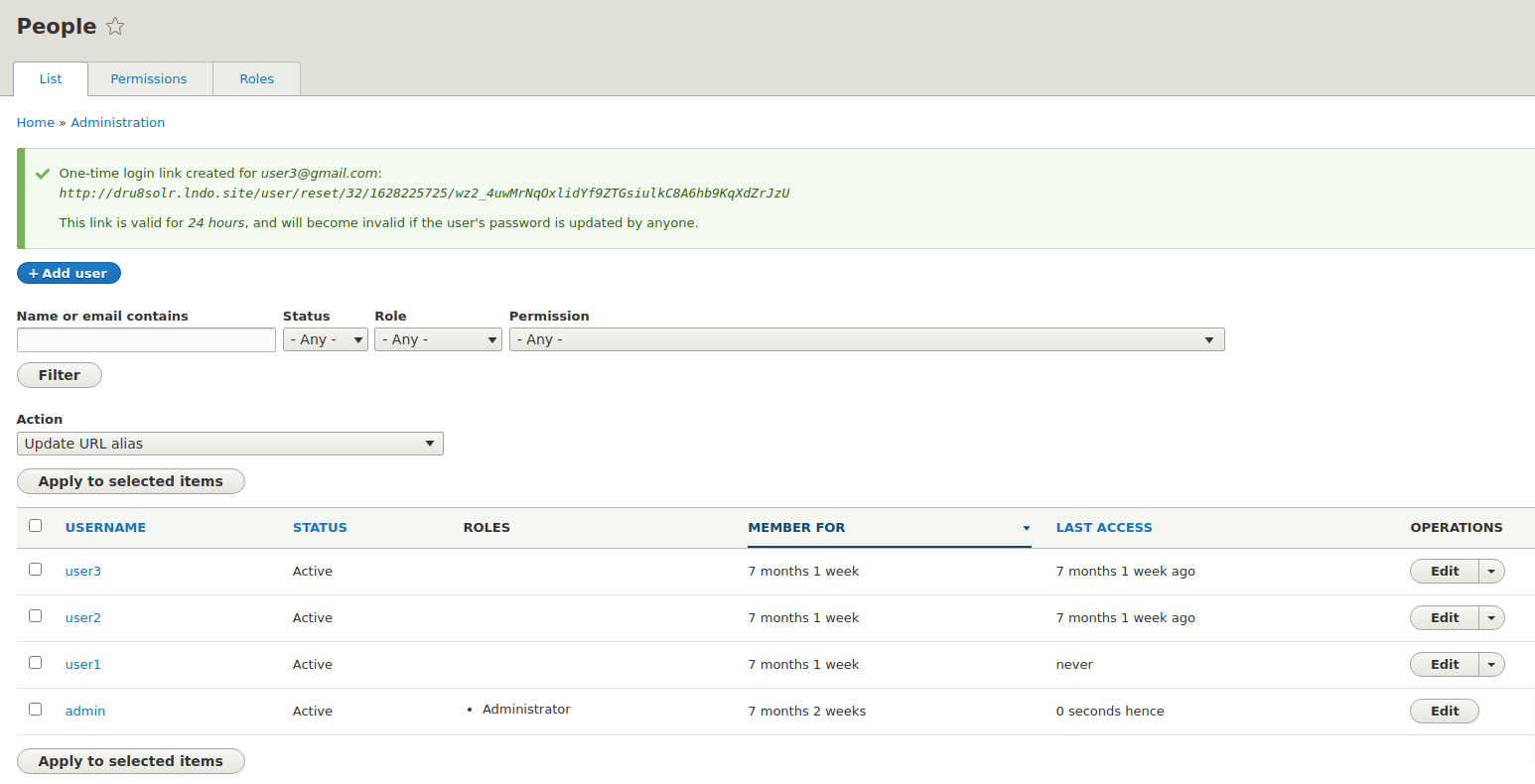The image displays an admin panel with several distinctive elements. At the top, a gray bar extends across the entire width of the screen, prominently featuring the word "People" in black, accompanied by a light gray star icon. Below this header, there are three tabs labeled "List," "Permissions," and "Roles." The "List" tab is selected and highlighted in white, while the "Permissions" and "Roles" tabs are in pink with blue text.

Underneath these tabs, the navigation options "Home" and "Administration" are visible. A significant feature on this panel is a one-time login link generated for the email user3.gmail.com. This link is notably large and is valid for 24 hours, becoming invalid if the user's password is updated by anyone.

There is a blue capsule button labeled "Add User," next to a field designated for entering a name or email that matches specified criteria. Additional filter options include "Status," "Role," and "Permission," with default settings set to "Any" but allowing for selections from drop-down menus. A button labeled "Apply Filter" is also available.

Toward the bottom, there is a drop-down menu under "Action" for updating the URL alias, with an "Apply to Selected Items" button adjacent to it. The user table is organized into columns: "Username," "Status," "Roles," "Member For," "Last Access," and "Operations."

- Under "Username," the list includes user3, user2, user1, and admin.
- In the "Status" column, all users are marked as active.
- The "Roles" column shows that only the "admin" user has the role "Administrator," whereas the others are blank.
- The "Member For" column indicates that user3, user2, and user1 have been members for seven months and one week, whereas the admin has been a member for seven months and two weeks.
- The "Last Access" column shows varying access times: "seven months and one week ago" for user3 and user2, "never" for user1, and "0 seconds hence" for the admin.
- The "Operations" column provides an "Edit" button with a drop-down menu for the top three users and a simple "Edit" button for the admin.

At the bottom left corner, there is another button labeled "Apply to Selected Items" in a blue capsule format.